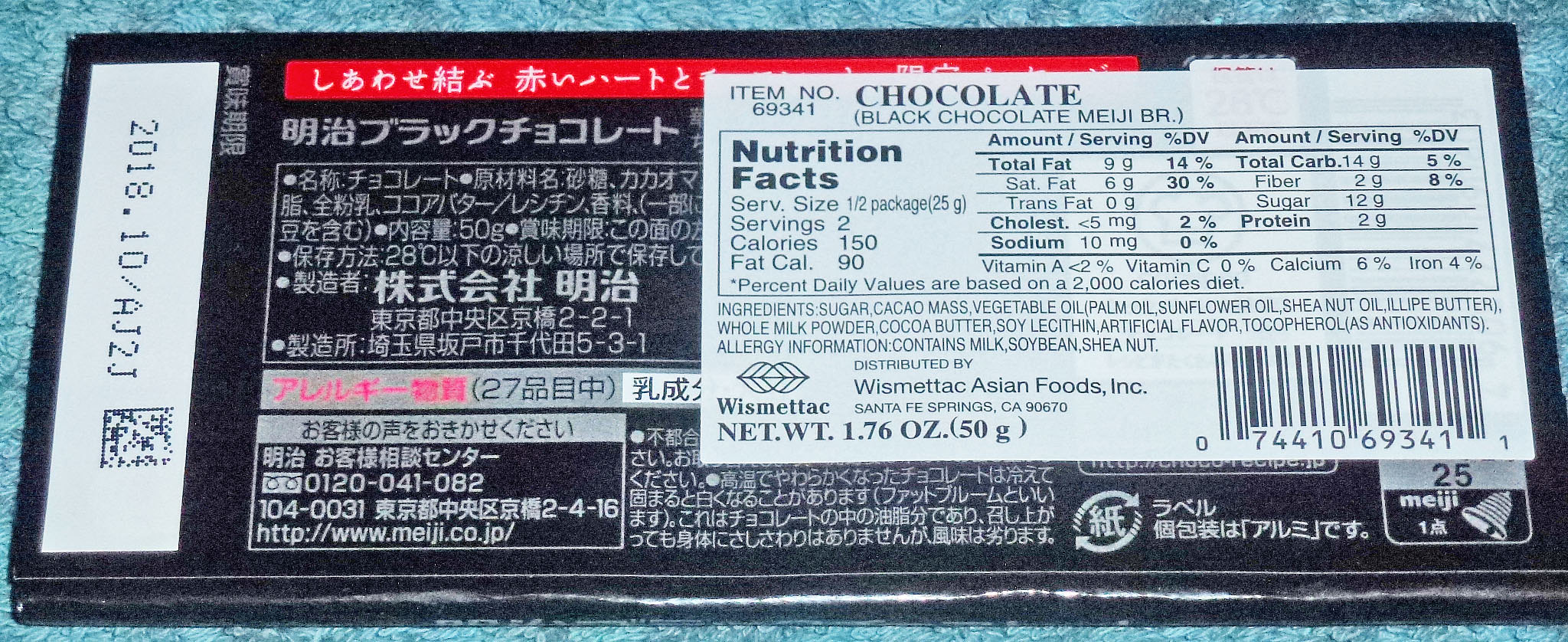This image showcases the back side of a Japanese chocolate bar, identified as a Meiji black chocolate bar. The packaging is primarily in Japanese kanji, with an additional sticker providing English translations. The expiration date, marked on the left side, is 2018-10. To the top right, there is a Nutrition Facts label stating the details for "chocolate, black chocolate Meiji bar," indicating 9g of total fat, 6g of saturated fat, 0g of trans fat, and a calorie count of 150 per serving, with the product serving two portions. Detailed ingredient information includes sugar, cocoa mass, vegetable oil, milk powder, cocoa butter, soy, and artificial flavor, and it is produced by Wismed Tech Asian Foods Inc.